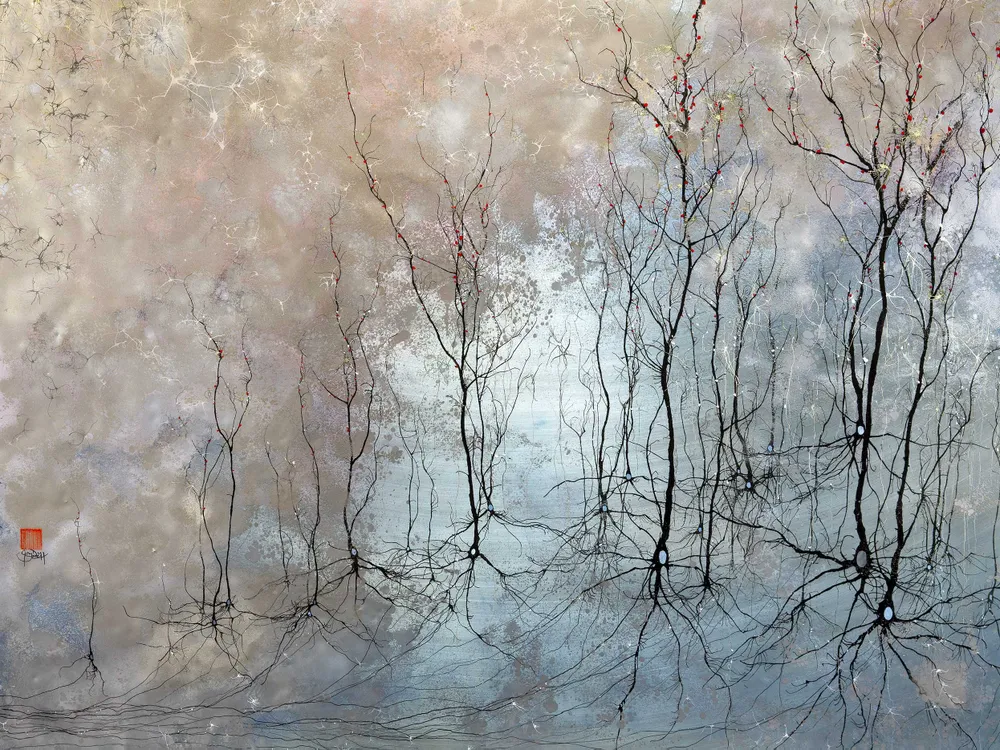This image captures an abstract watercolor painting with intricate details. The painting features thin, black, wispy trees with visible roots, making them appear almost like delicate vines sprouting from a powder blue, desolate lake. The trees seem devoid of leaves, and their reflections can be seen in the murky water. The upper sections of the artwork exhibit light tan marbling, blending with patches of blue, reminiscent of a sky peeking through the trees. Nestled within this scene are specks of blue, yellow, and perhaps red, resembling berries. There are also small blue and gray details that seem to hang or button onto the spindly branches. The left side of the painting houses a tiny red mark with black writing—an artist’s signature, though too small to decipher clearly. The overall effect is like peering into a serene, mystical woodland pond encased by branches under a pale blue sky.